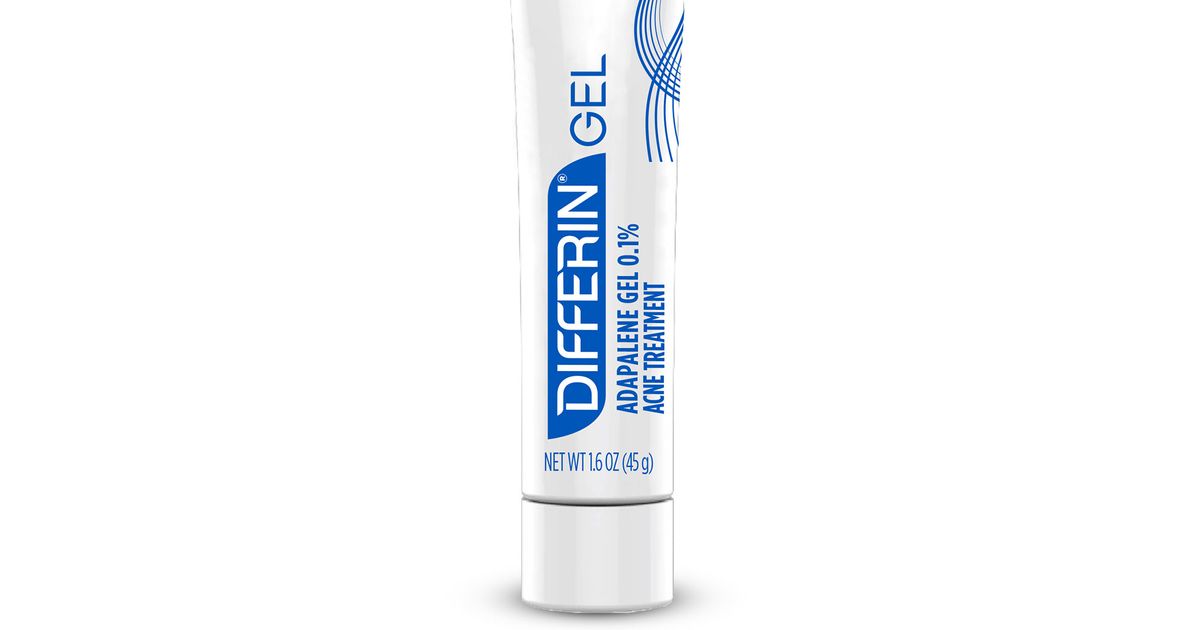The image showcases a white cylindrical tube of Differin gel placed against a plain white background. The tube features text in royal blue, arranged vertically along its length, reading "Differin gel Adapalene gel 0.1% Acne Treatment." At the bottom of the tube, aligned horizontally and perpendicular to the other text, it indicates "Net Weight 1.6 oz (45 grams)." The Differin logo is highlighted in white letters atop a blue, swirling design located in the top right-hand corner. The tube is capped with a smaller white cylindrical lid, approximately one-fifth the size of the tube, and is positioned at the base.